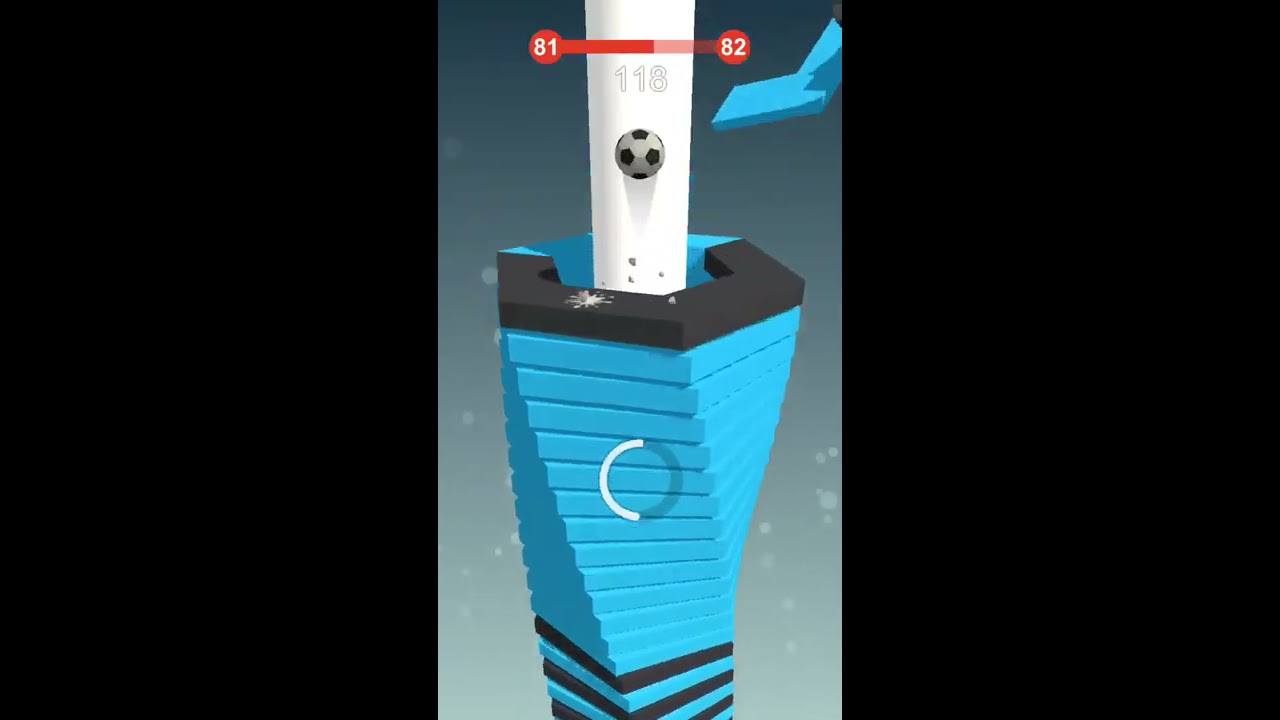The image appears to be a screenshot of a video game screen, primarily featuring a central white pillar surrounded by a hexagonal tube that spirals and curves upwards. The left and right portions of the screen are black, creating a focused view on the central gameplay area. At the top of the screen, a red bar transitions from a darker to a lighter shade, connecting the numbers 81 and 82, which may represent levels or scores. Below this, the number 118 is prominently displayed, possibly indicating the player's score.

A soccer ball is positioned in the middle, seemingly interacting with the pillar and the hexagonal shapes. These hexagons alternate between blue and black, forming a pattern that extends downwards for about 15 stories. The top section of the hexagon structure is blue, while the other three sides are black in color. Additionally, there are colorful paint splashes at various points, including the bottom left and right of the hexagon tower. A blue paddle-like object extends from the right corner, adding another interactive element to the scene. The overall composition of this image, including the alternating colors and the centrally positioned soccer ball, suggests dynamic gameplay mechanics.